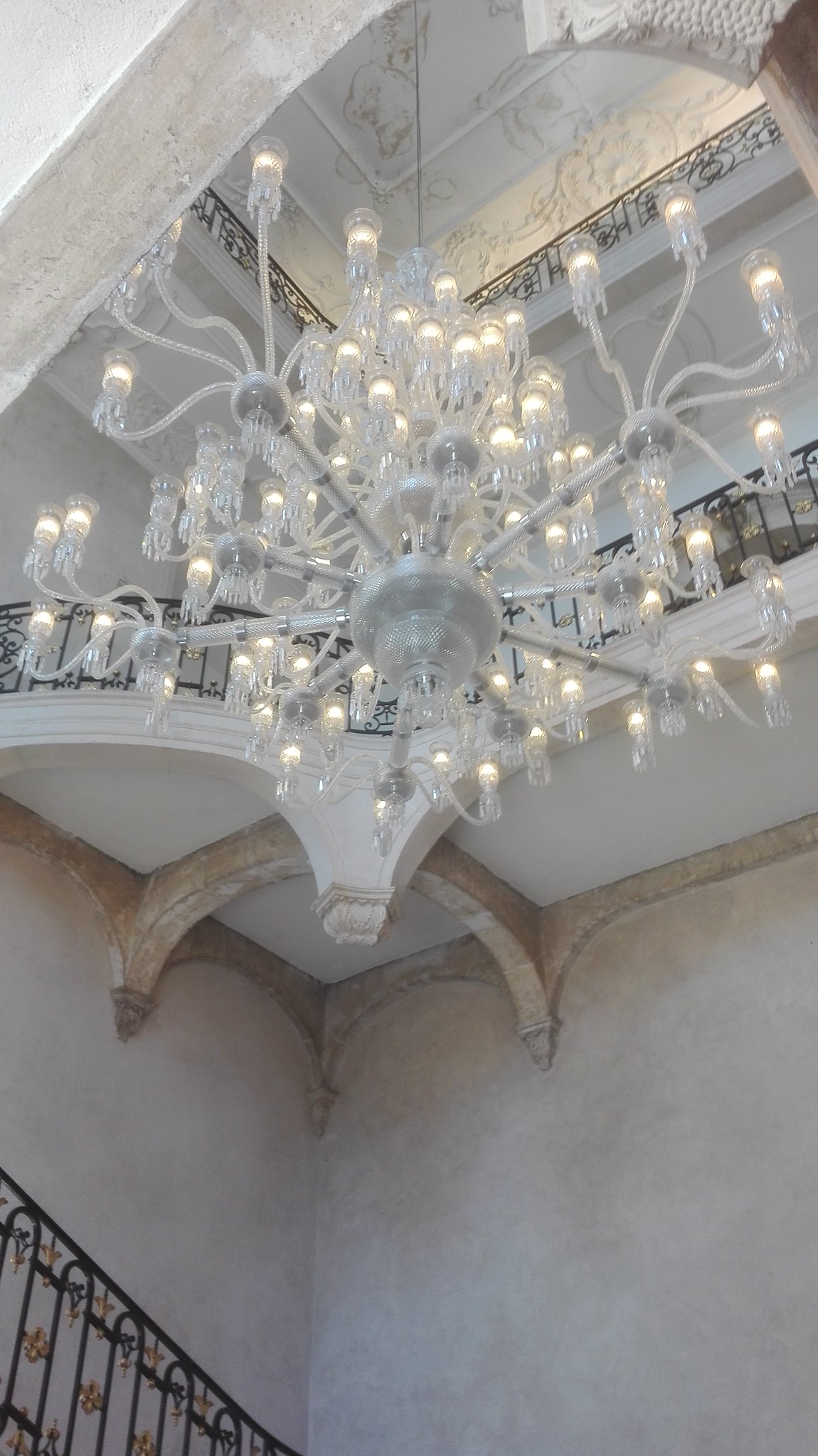This color photograph, displayed in portrait orientation, captures the interior of a large, elaborately designed stone structure. Central to the image is an ornate white chandelier with numerous arms, each adorned with candle-like lights, crystal teardrops, and intricate facets that lend it a shiny, Gothic appearance. The chandelier is illuminated and suspended from a ceiling adorned with white ornamental molding and decorative motifs. Surrounding the chandelier, black wrought iron stairwells and balconies with elaborate carvings and gold fleur-de-lis ornaments create a tiered, balconied effect, giving a sense of depth as they ascend upwards. The photograph suggests a view from a lower level, possibly a staircase, looking up at this grand architectural feature. The overall ambiance of the building is light, with elements of white plaster and old wood molding contributing to its historical and sophisticated atmosphere.